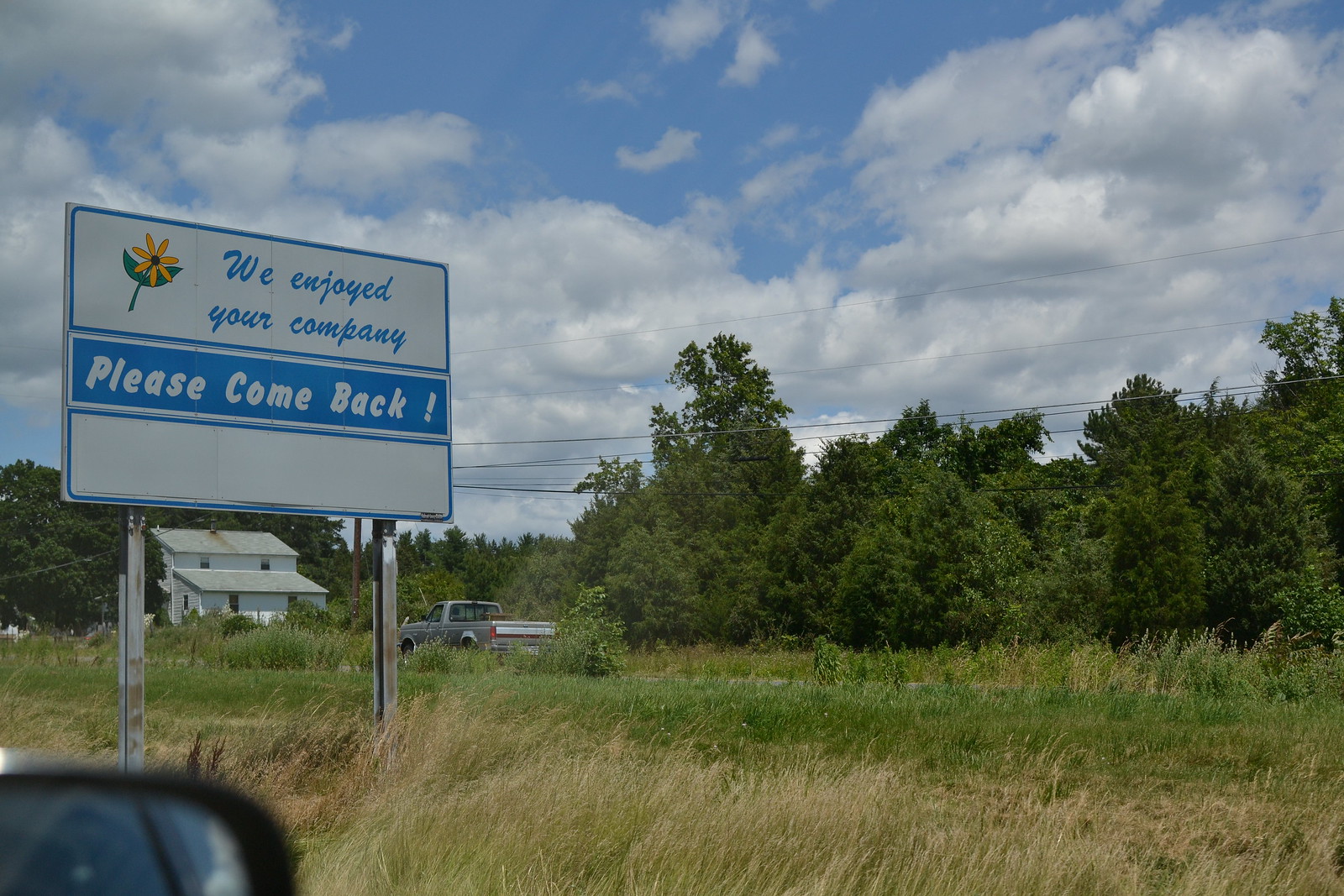The photograph captures the serene view from inside a car, looking out through the window. In the bottom left-hand corner, the side mirror is visible. The scene outside is bathed in natural light, showcasing tall grass and distant trees under a vivid blue sky dotted with large, fluffy white clouds. Prominently featured in the mid-ground is a white and blue road sign with a yellow flower, which warmly reads, "We enjoyed your company, please come back," though it doesn’t specify the location.

Further back, a gray pickup truck is parked near the sign, adding to the rural ambiance. To the right of the sign stands a quaint, white two-story house, contributing to the picturesque, bucolic setting. Power lines stretch horizontally across the image, cutting through the open space and emphasizing the rural landscape.